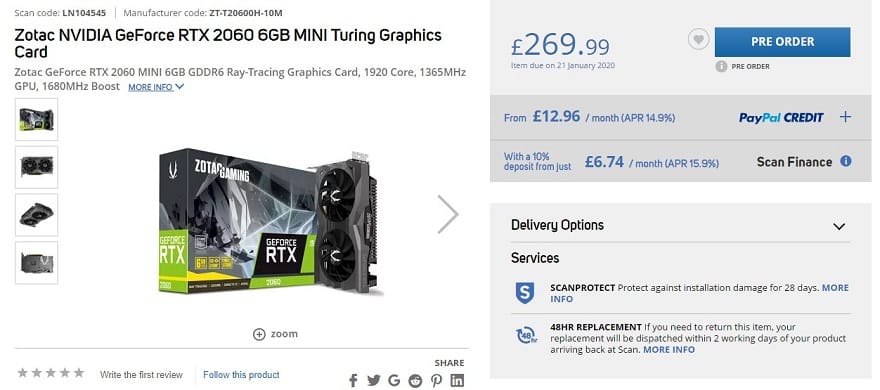**Zotac GeForce RTX 2060 Mini Graphics Card**

Introducing the compact yet powerful Zotac NVIDIA GeForce RTX 2060 Mini graphics card featuring 6GB of GDDR6 memory. This exceptional Turing architecture-based GPU supports advanced ray tracing technology for stunning visual effects and lifelike graphics. Ideal for high-performance gaming or intensive graphic applications, the RTX 2060 Mini offers superior performance in a small form factor.

**Product Details:**
- **Model:** CT-T20600H-10M
- **Memory:** 6GB GDDR6
- **Architecture:** Turing
- **Ray Tracing Support:** Yes
- **Replacement Policy:** 48-hour replacement if needed, with dispatch within 2 to 3 days upon item return and scan.
- **Scan Code:** LN104545

Designed to fit in mini-ITX cases without compromising on power, this graphics card ensures you get the best gaming experience in a smaller package. Return or replacement processes are efficient, providing peace of mind with a quick turnaround.